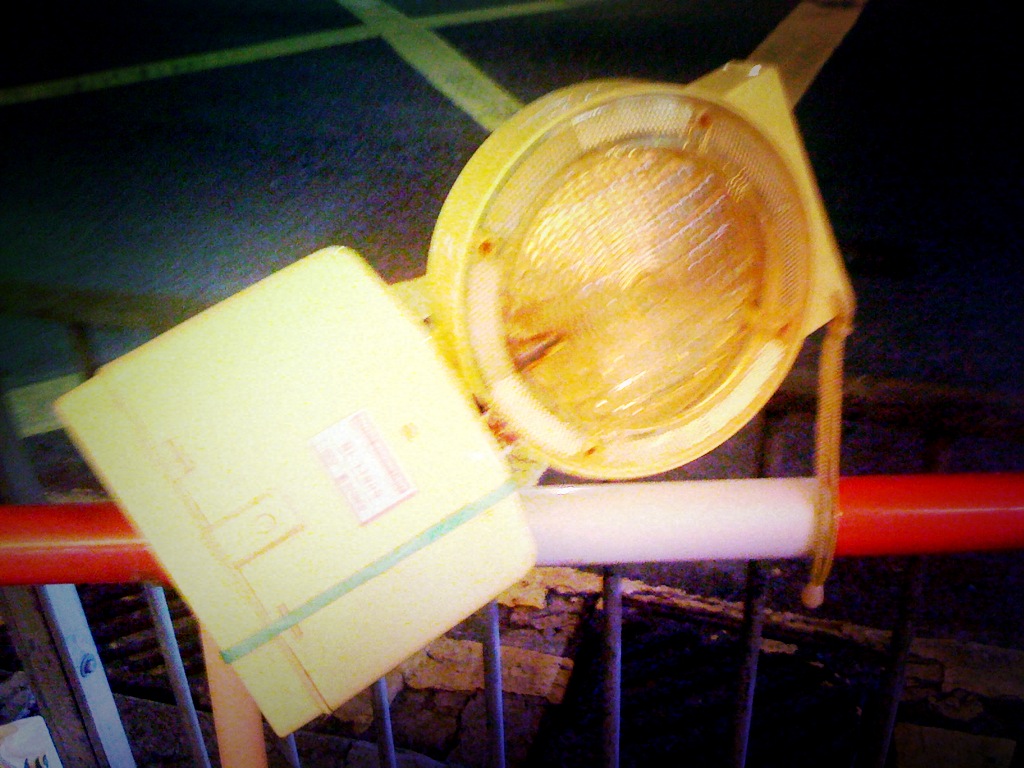The photograph captures a nighttime road construction safety light in detail. The base of the light is a sturdy, yellow plastic cube, which serves as a foundation for stability. This base is cinched by a green rubber band wrapped securely around it. Sitting atop the cube is a circular yellow plastic disc, designed with a specialized lens that emits a flashing yellow light. This light serves as a critical visual indicator for drivers, signaling ongoing road work or construction ahead. In the background, yellow lines painted on the road add context to the setting, underscoring the structured guidelines of the construction area.